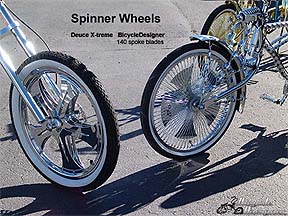This horizontally oriented, realistic photograph showcases a detailed close-up of chrome spinner wheels on bicycles. The image, likely an advertisement, prominently features the title "Spinner Wheels" along with "Deuce Xtreme Bicycle Design and 140 Spoke Blades" in black font. These fancy, aesthetically focused wheels bear shiny chrome and white sidewalls, indicating their premium nature over everyday use wheels. The scene captures the bikes parked on a street-like pavement in bright daylight, casting pronounced shadows from the wheels. In the foreground, the front wheel of a bike on the left is distinctly visible with black rubber and chrome spinners, while a similar wheel with a slightly smaller spinner is seen on the right. Additionally, another front bike tire appears in the background. The image also includes an indistinct business logo at the bottom corners, reinforcing the promotional intent of these high-end bicycle components.